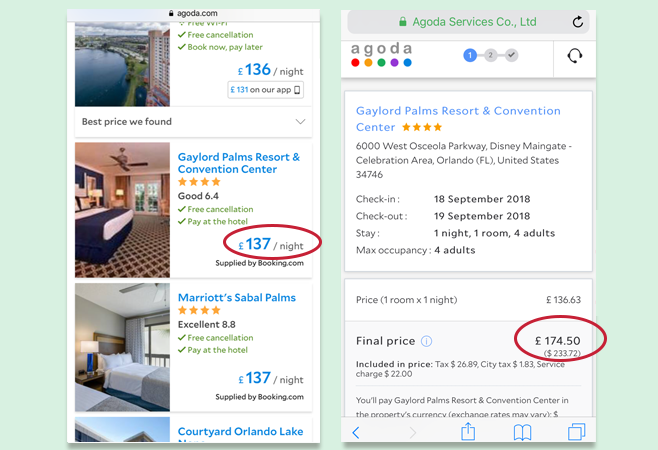This image displays two adjacent mobile-optimized web pages from Agoda.com, framed against a green background. Both pages have a white backdrop, and the primary content appears to focus on hotel bookings.

On the left page, the header shows the Agoda logo alongside a padlock icon, indicating a secure site. A striking photograph of tall buildings beside a serene lake or sea serves as the visual centerpiece. Prominent text beside the image advertises "Free cancellation, book now, pay later," with pricing noted at £136 per night, reduced to £131 through the app – emphasized as the best available rate. Below, listings for hotel rooms include detailed descriptions and images of the accommodations. 

- **Gaylord Palms Resort and Convention Centre**: Features a bedroom image on the left with a rating of 4 stars and a score of 6.4, described as "Good." Free cancellation is mentioned, with an option to pay at the hotel. The rate is set at £137 per night, highlighted by a red oval. 
- **Marriott Sabal Palms**: Displays a similar layout with an "Excellent" rating of 8.8. The nightly rate is the same at £137, accompanied by a bedroom picture.

The lower part of the left page partially shows another listing titled "Cortland Orlando Lake."

The right page centers around a search interface, labelled "Agoda Services Co Ltd". Below, the Agoda logo appears with five multicolored circles (red, orange, green, purple, blue). Checkboxes indicate steps or options, with "1" currently highlighted in blue.

Further details for Gaylord Palms Resort and Convention Centre are provided:

- Address: 600 West (partial)
- Check-in Date: 18 September 2018
- Check-out Date: 19 September 2018
- Duration: 1 night
- Room Occupancy: 1 room for 4 adults, maximum occupancy
- Room Rate: £136.63 per night

The final total is £174.50, broken down as:

- Tax: £26.89
- City Tax: £1.83
- Service Charge: $22

The final price is calculated for payment directly to Gaylord Palms Resort and Convention Centre at the property's currency exchange rate. Three blue icons and a black arrow appear beneath this information, indicating navigation or additional options.